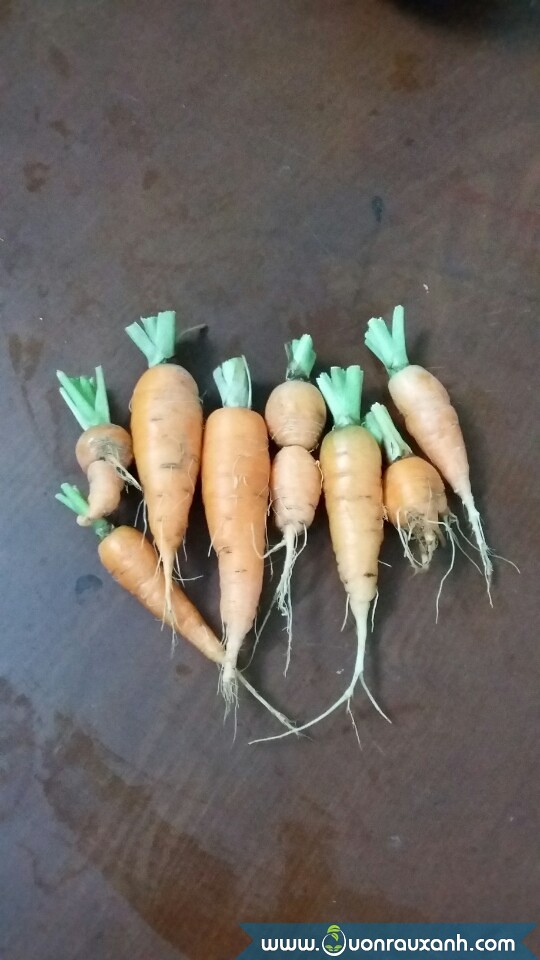This is a detailed overhead photograph showcasing a group of eight unusually shaped homegrown carrots arranged on a dark brown, slightly dusty wooden table with visible moisture streaks. The carrots, exhibiting a pale to light orange hue, are aesthetically complemented by an inch or two of light green stems at their tops. Each carrot features distinct characteristics: some have petite, almost ping-pong ball-like forms, while others are elongated or display curious double-circle shapes. Fine hair-like roots dangle from their ends, enhancing their homegrown charm. The centerpiece includes one carrot with a unique double-rounded shape. An additional carrot lies diagonally below the main row. At the bottom left corner, a blue banner with white text reads "www.vonrauxanh.com," further detailing the image.